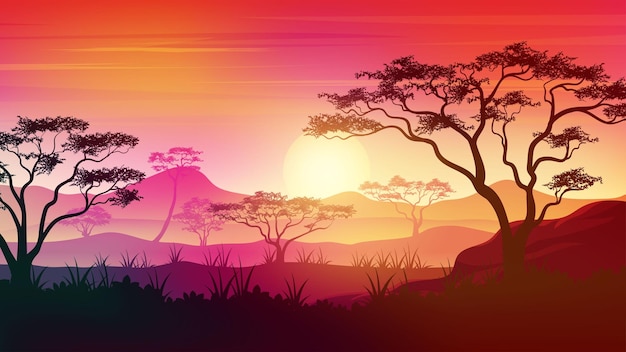The image is a computer-generated drawing of a cartoony desert landscape during a sunset. The sky is a blend of reddish yellow, orange, and purple hues, with the sun prominently displayed on the horizon. The trees, which are silhouetted and sparse with long, winding branches and scattered leaves, frame the scene on both sides. The landscape features a series of rolling hills that recede into the distance, with various shapes and shades of orange. In the foreground, small blades of grass emerge from the sandy terrain, also appearing as silhouettes. The overall scene resembles a vibrant wallpaper with its blend of vivid colors and digital artistry.